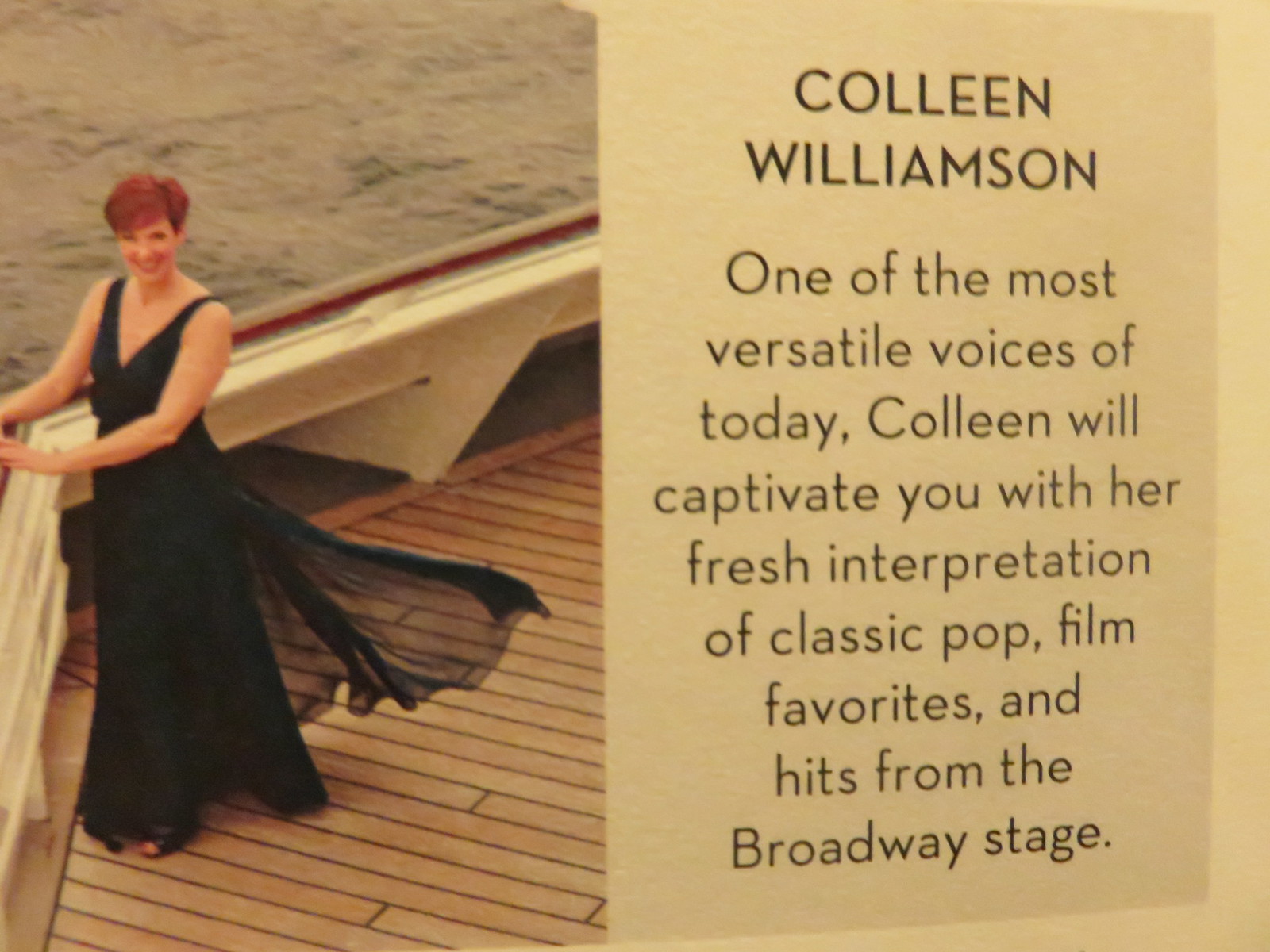The image features a white-bordered placard photographed at an angle, making the right side appear slightly smaller than the left. The placard is divided into two sections. The left section showcases a photograph of a woman, identified as Colleen Williamson, standing on a boat. Colleen, a middle-aged, white woman with short red hair, is smiling warmly at the camera. She is dressed in a black sleeveless evening gown with a low V neckline that reveals a hint of cleavage, and a sheer black train billows gracefully at the back of her dress. Her hands rest elegantly on the white railing of the boat, which is set against a backdrop of smooth wooden planks and a serene water scene. The right section of the placard is a gray rectangle bearing black text that reads: "Colleen Williamson. One of the most versatile voices of today, Colleen will captivate you with her fresh interpretation of classic pop, film favorites, and hits from Broadway stage."